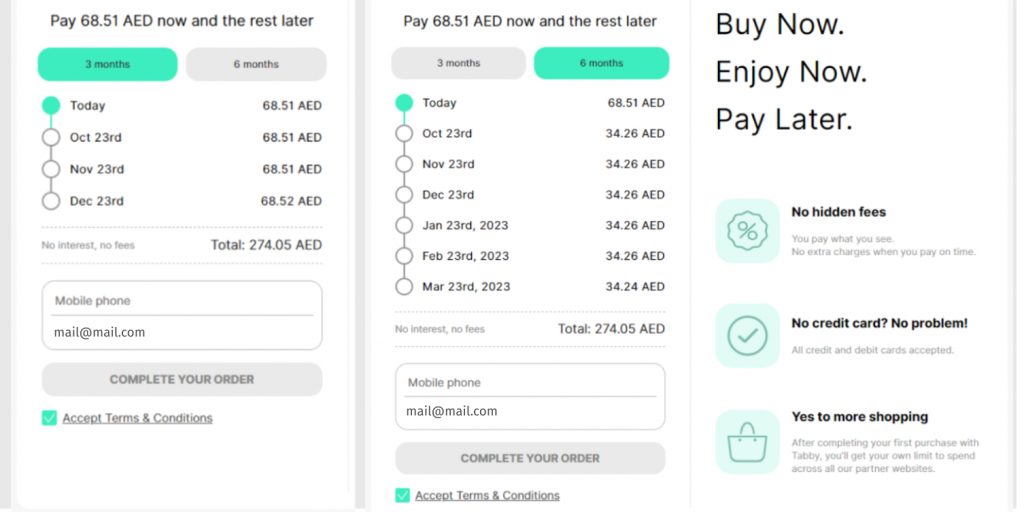This image captures a smartphone display showcasing a payment plan selection screen. It appears to be a composite of three separate screenshots arranged side by side, providing a detailed comparison between different payment plan options.

On the left screen, the interface prompts the user to "Pay 68.51 AED now and the rest over the year." The selected payment plan is highlighted by a green button indicating a three-month installment period. 

In the middle screen, the same prompt is shown, but this time with the six-month installment option highlighted in green, while the previously selected three-month option has reverted to gray. Both the three-month and six-month options feature a "Pay Today" button, marked with a green dot, and a green checkmark next to "Accept terms and conditions."

The far-right screen displays a summary page with the message "Buy now, enjoy now, pay later." It reassures the user with phrases such as "No hidden fees," "No credit card? No problem," and "Yes to more shopping," emphasizing convenience and affordability.

The image effectively showcases the payment flexibility and ease offered by the application, with visually distinct indicators like green buttons and checkmarks enhancing the user experience.